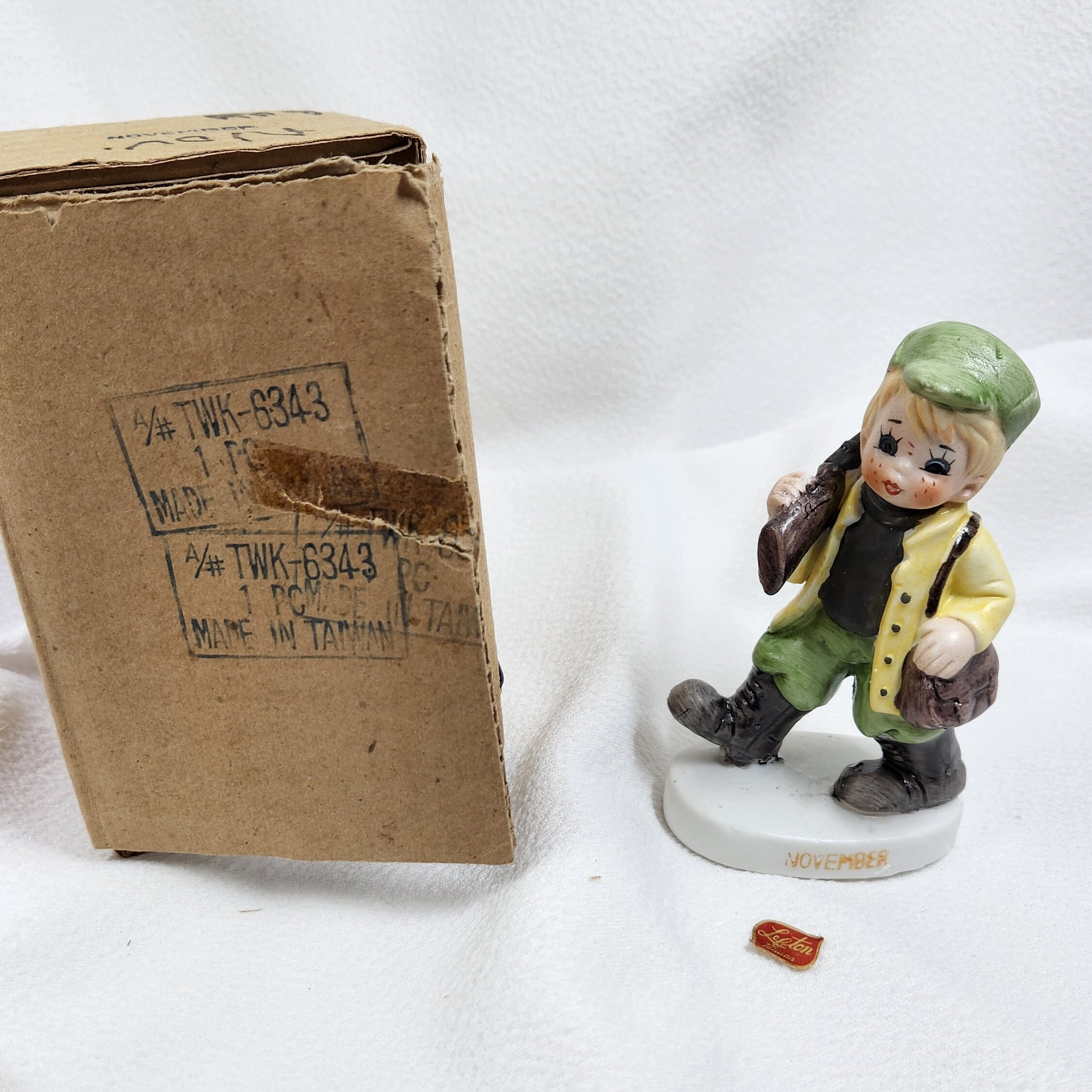The image features a detailed photorealistic scene of a porcelain figurine and a cardboard box set against a white textured cloth backdrop. The figurine is positioned on the right and portrays a young boy, dressed as a hunter, complete with blonde hair, large blue eyes with exaggerated eyelashes, and rosy cheeks adorned with freckles. He wears a yellow jacket with black buttons, a black turtleneck, sage-green pants, and black boots. A green cap sits atop his head, and he carries a rifle slung over his left shoulder and an ammunition bag on his right. The boy sits on a white circular pedestal inscribed with "November."

In front of the pedestal, a small red label, possibly original to the piece, is visible but unreadable. The cardboard box, appearing worn and partially torn, sits on the left side of the image. The box has three visible stamps, including "Made in Taiwan," "One Piece," and "TWK-6343." The box's top is slightly open and shows signs of repair with tape. The overall setup, including the white cloth backdrop, suggests the image may have been arranged to highlight certain features or possible damage to the items. A notable point is a small red sticker in front of the statue, which might be a piece of the original packaging or a sales label. The sticker also includes the word "Lepton," likely indicating the brand of the figurine.